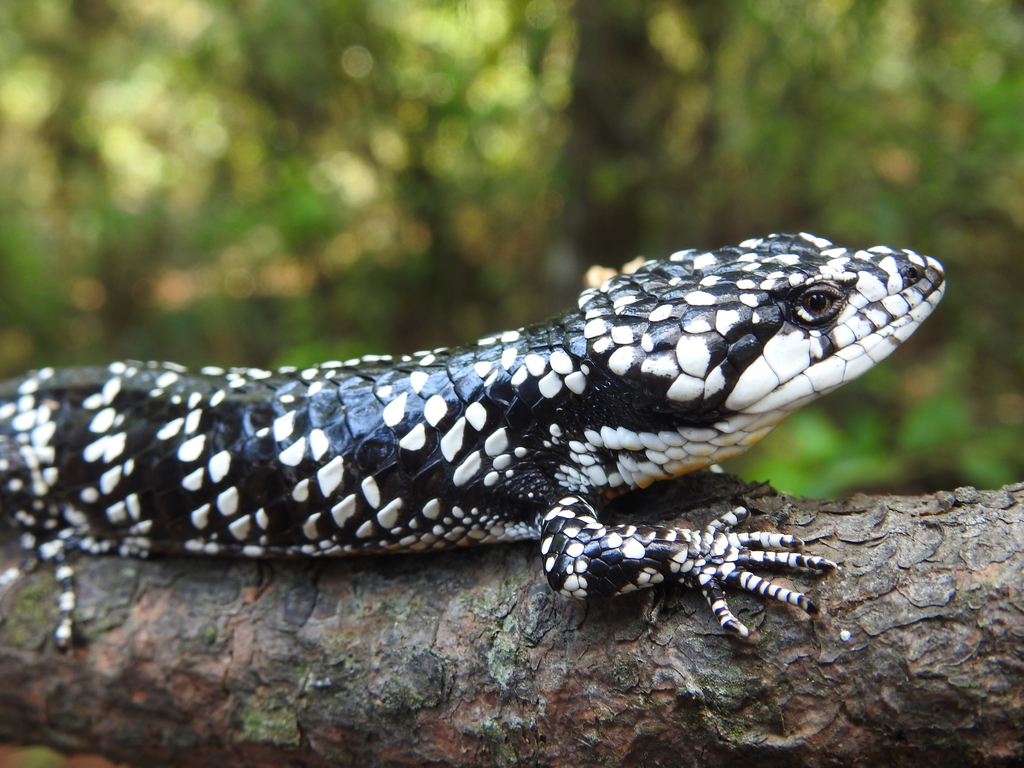The image captures a detailed scene of a black and white salamander perched on a wide tree branch in a brightly lit forest setting. The salamander resembles a small lizard and is prominently highlighted against a blurred green and yellow background, suggesting a forest environment. The branch it rests on, grayish with patches of orange bark, spans the bottom third of the image.

The salamander's distinctive markings are notable: it has a predominantly white underside with black and white triangle-shaped scales, which give it a striking appearance. The head, turned towards the right side of the image, reveals one eye looking straight at the camera. Its face features a white area around the mouth, with black markings around the nose extending over the head and along its body. The front leg and partial hind leg with toes are visible, though not the entire back side.

The photograph is crisp and clear, taken during the daytime with ample natural light, focusing sharply on the salamander and branch, while the forest background remains softly blurred.